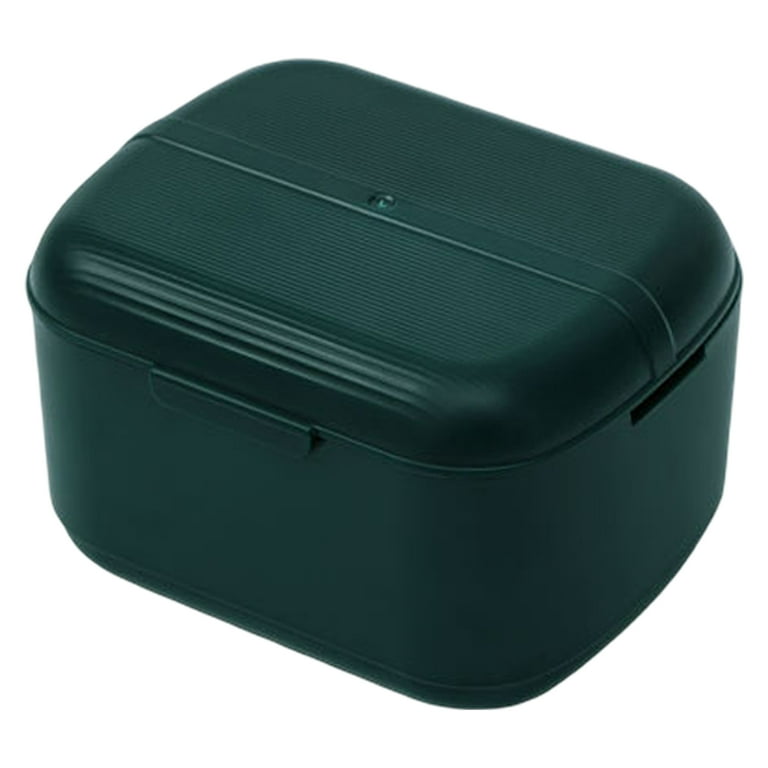This photograph features a green plastic case that is slightly elongated compared to a cube, with smooth, rounded edges and no sharp corners. The case's bottom half is unremarkable, being dark gray in color and entirely smooth. The top lid of the case, a darker shade of green, is ribbed, except for a smooth band stretching across its length. At the center of this band is a small, circular indention, possibly a screw or rivet. The lid snaps securely onto the case with plastic latches on either side. Additionally, there is a small vent near the top edges of the case, not covered by the lid. The image of the case appears to be isolated, with no visible background.